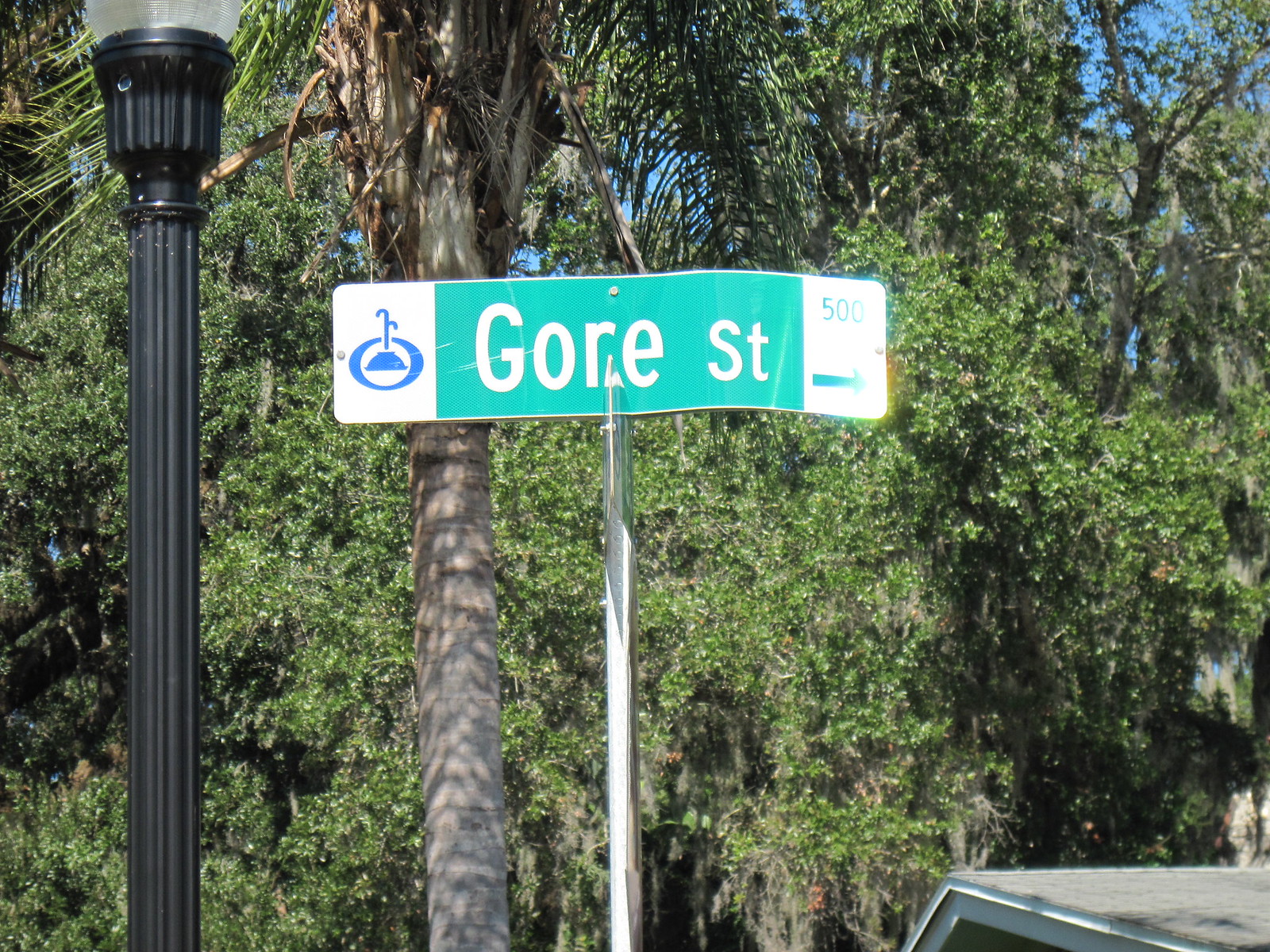This image captures a detailed view of a street intersection marked by distinct signage. Two green and white banner-type street signs are mounted on black posts. The foremost sign, centered in the image, reads "Gore ST" in white letters against a green background. Below, a white panel on the right side shows the number "500" alongside a green arrow pointing to the right, while a white panel on the left displays a blue circular icon resembling a fountain or plant emerging from an inverted bowl shape. The second sign is positioned such that the camera view is parallel to its thin edge, rendering its text unreadable but still visibly present. Adjacent to the signs, a black street lamp with a glass top rises against a backdrop of lush green trees and glimpses of blue sky peeking through the foliage, creating a picturesque and informative snapshot of this urban locale.